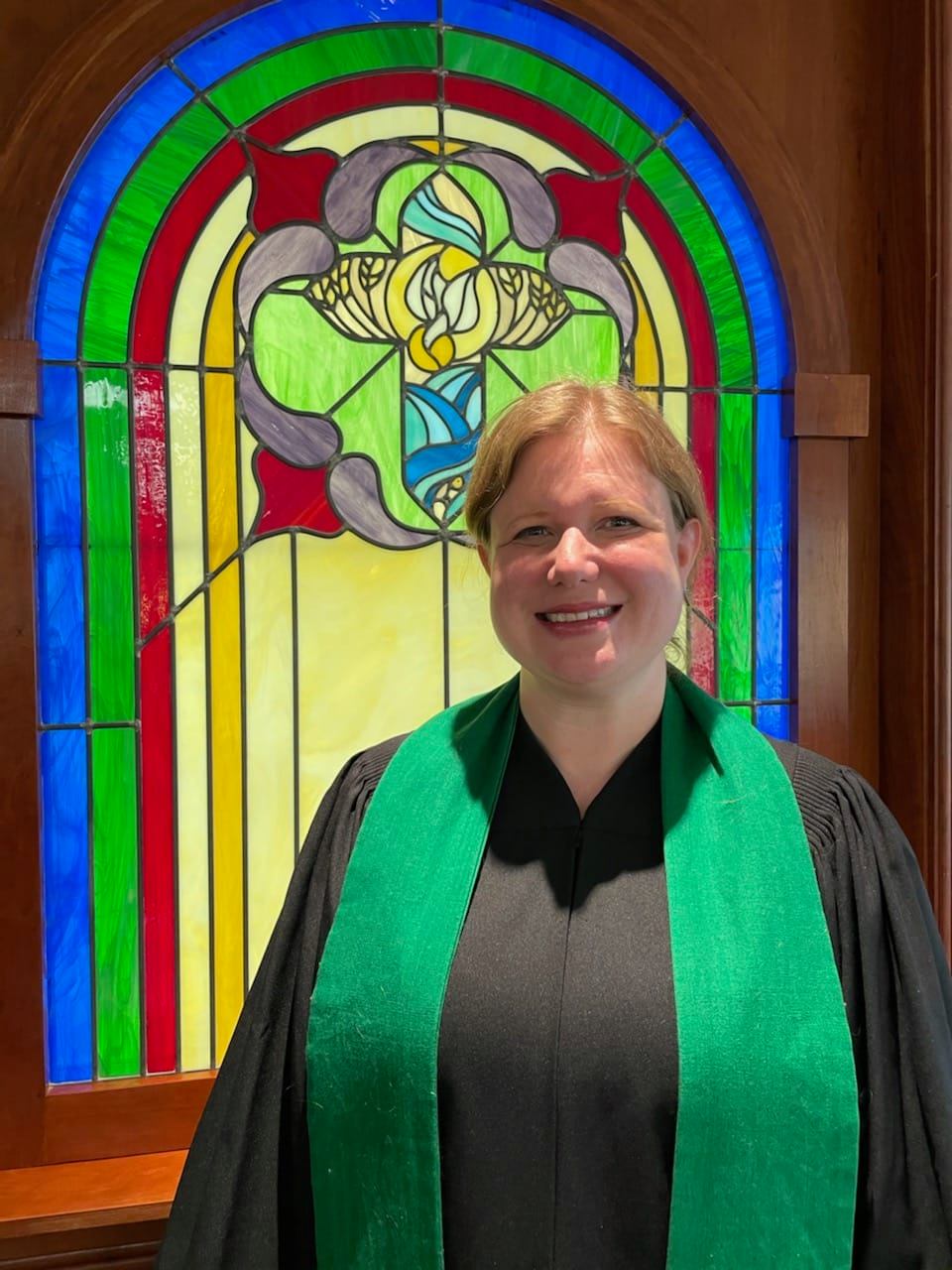This is a photograph of a middle-aged blonde Caucasian woman, possibly a religious figure or choir singer, standing in front of an arched stained glass window. She has light brown hair and a plump build, with a warm smile directed at the camera. She is dressed in a black robe with a shallow V cut at the neck, complemented by a green stole draped over her shoulders, running along her entire left and right sides. The elaborate stained glass window behind her features a vibrant array of colors in a striped pattern: blue, green, red, light yellow, and dark yellow. At the center of the window is a cross, surrounded by a depiction of a river and a dove. Additionally, at the top of the arched window, there is a flower with yellow, green, purple, and red petals. This serene and ornate setting emphasizes the woman's likely connection to her religious congregation or choir.